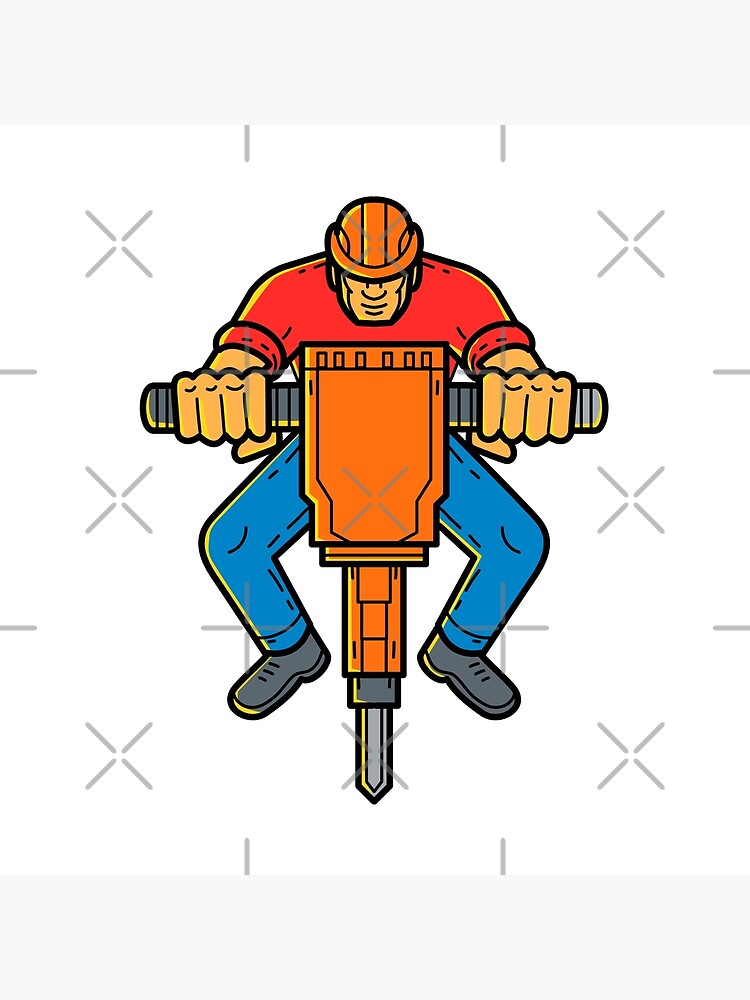The image is a cartoon graphic depicting a construction worker engaged in jackhammering. The worker, positioned against a white background adorned with grey X's and lines, is crouching with his knees bent as he operates a large, orange jackhammer. He is dressed in a red long-sleeved shirt rolled up to his elbows, blue jeans, and black or grey sneakers tinged with yellow. An orange safety hard hat covers the top of his head, and only the lower portion of his face—his nose, mouth, and chin—is visible. The jackhammer, held by two sidebars with vertical lines and a yellow tinge, is striking an indeterminate, vector-themed ground surface. This type of image is typically used for graphic design projects such as posters, flyers, or websites.